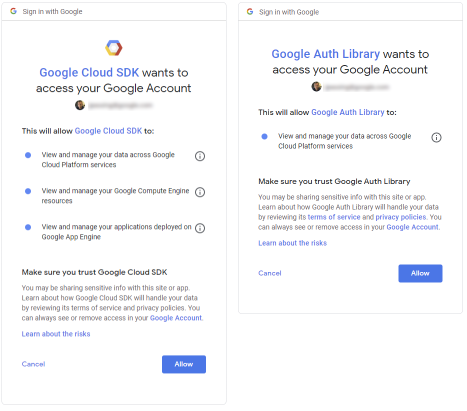The image depicts two distinct permission request screens, likely originating from a mobile device due to the portrait layout of the separate rectangles. Both screens are designed to appear as "Sign in with Google" dialogs.

The first screen displays a prompt from "Google Cloud SDK," seeking authorization to access the user's Google account. At the top, the familiar Google logo lends authenticity, followed by a section where the user's profile picture and account name are shown but intentionally obscured. The request explicitly outlines three specific permissions it intends to obtain. Users are cautioned to ensure they trust "Google Cloud SDK" and are presented with options to either "Cancel" or "Allow" the request, with the "Allow" button prominently highlighted in blue.

The second screen mirrors the layout and design of the first but pertains to "Google Auth Library." Similarly, it asks to view and manage the user’s data across Google Cloud Platform services. The user's profile picture and account name remain obscured for privacy. This screen also provides a reminder to verify trust in "Google Auth Library" before granting permissions. As with the first screen, users can choose between "Cancel" or "Allow," with the latter again highlighted.

Overall, these screens illustrate the steps involved in granting apps access to a Google account, emphasizing user caution and the importance of understanding the permissions being requested.